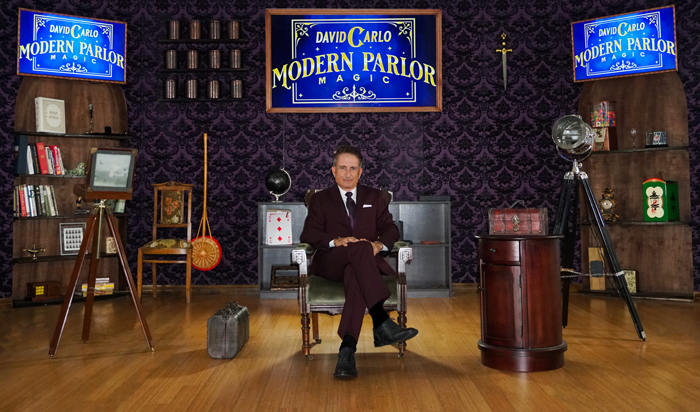The image showcases a detailed and somewhat vintage scene of a modern parlor magic stage set with a man seated at its center. Identified by a large blue sign bordered in wood above him, labeled "David Carlo, Modern Parlor Magic," this man appears to be David Carlo, potentially a magician, dressed in a dark, burgundy suit with black shoes and socks. He has brown hair and is seated with his right leg crossed over his left, hands resting on his knees in an upholstered chair with greenish fabric and wooden arms. The background is adorned with a dark gray, diamond-pattern wallpaper.

The stage is intricately decorated with various objects. To the right, there's a wooden bookshelf containing books, a statue, a trophy or candlestick, and an old radio. Above the bookshelf are vintage cans arranged in rows of four, presumably for shooting practice, and a small dagger hangs on the wall. There's also an old chair with a floral pattern, an antique camera on a wooden tripod, and a black spotlight on a tripod stand.

On the left side of the stage, another matching bookshelf holds more books, a gumball machine, an old clock, an indistinct green object, and a reddish treasure box atop a small round table. Near the man's chair lies a gray suitcase or bag, and a metal shelf behind him displays additional items including a large playing card and a black globe, enhancing the magical ambiance of the setting. 

The floor of the stage is a polished hardwood, completing the elegant, nostalgic aesthetic of this intriguing modern parlor magic scene.